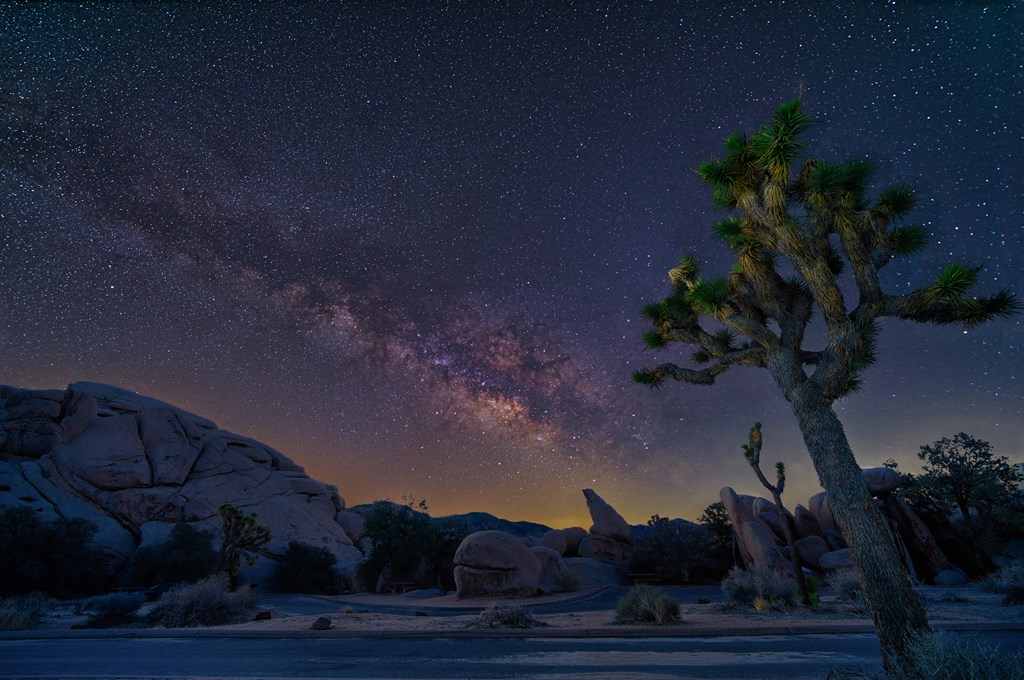In this captivating nightscape set amidst a desert environment, the scene could be either a highly detailed painting or a photograph. The sky, the central focus, is rich with stars and features a vivid band of the Milky Way stretching diagonally from the lower center, where remnants of a sunset bathe the horizon in blues and oranges, up towards the top left. The sky transitions into deep blues and purples, dotted with numerous white stars. At the base of the image, the landscape is subtly illuminated, revealing a terrain of sandy dirt interspersed with boulders and rocky formations, possibly resembling a giant boulder on the left. To the bottom right stands a distinctive, cactus-like tree, perhaps a Joshua tree, accompanied by smaller scrub shrubs. This natural desert scene is beautifully contrasted against the celestial spectacle above, where the nebula-like Milky Way adds an almost surreal, otherworldly dimension to the night.